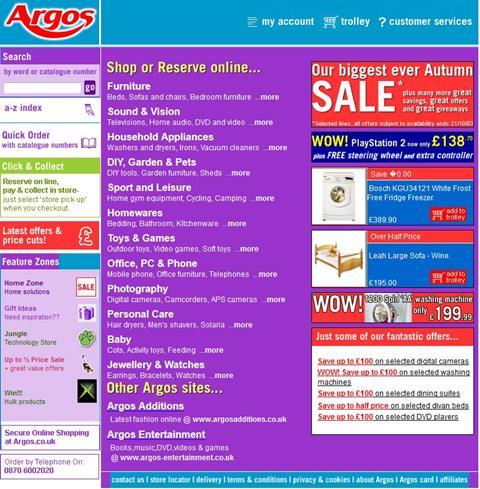Cropped screenshot of a vibrant and colorful website featuring prominent branding elements from Argos. At the very top is a blue banner, displaying the "Argos" logo in red letters on the left. Directly beneath the logo and still within the blue banner are links in small white text labeled "My Account," "Trolley," and "Customer Service." 

Below this blue banner, on the left side, sits a narrow, rectangular column with a purple background. At the top of this column, "Search" is displayed in the top left corner with a search bar below it, labeled "Keyword or Catalog Number." Proceeding downwards, the column features links titled "A to Z Index," "Quick Order," "Click and Collect" (highlighted in green), and a red banner with the text "Latest Offers and Price Cuts." Further down, another purple section labeled "Feature Zones" can be found.

The main content area to the right of this column has a purple background as well. It contains five small rectangular banners aligned vertically on the left side. Above these banners, there is a promotion for "Shopper Reserve Online." Following this, categories are listed vertically beneath, including "Furniture," "Sound and Vision," "Household Appliances," "Sport and Leisure," and "Toys and Games."